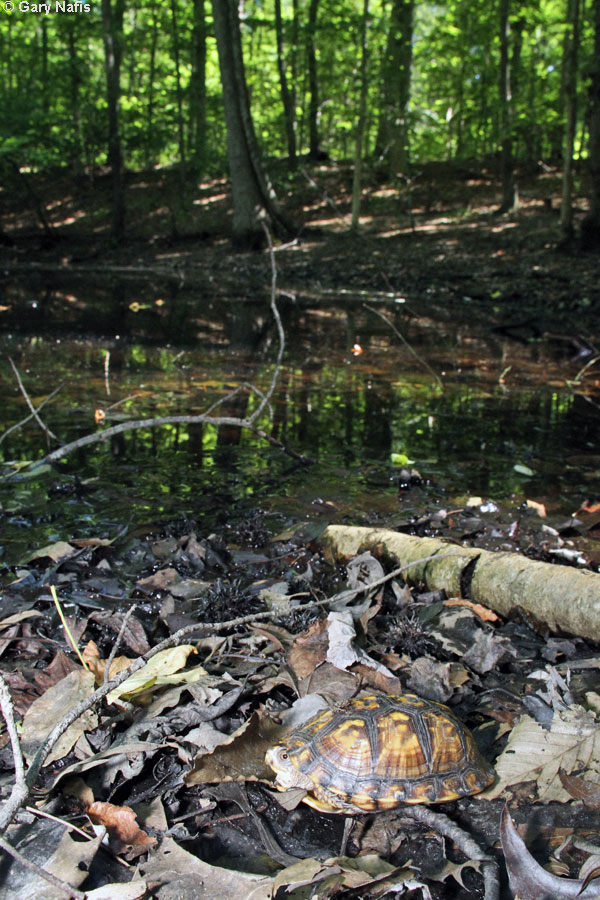In this outdoor photograph by Gary Nafis, a turtle is nestled among a bed of dead leaves, twigs, and small rocks, with a large log positioned on the right and a tree branch larger than the turtle itself to its left. The turtle, with a predominantly brown shell featuring dark markings and hints of black and yellow-orange, is partially hidden inside its shell. Its head is slightly extended, facing left, while its legs remain tucked in. This scene is set in front of a shallow body of water, possibly a creek or small lake, surrounded by a forest with a lush, green backdrop and a gentle upward slope.